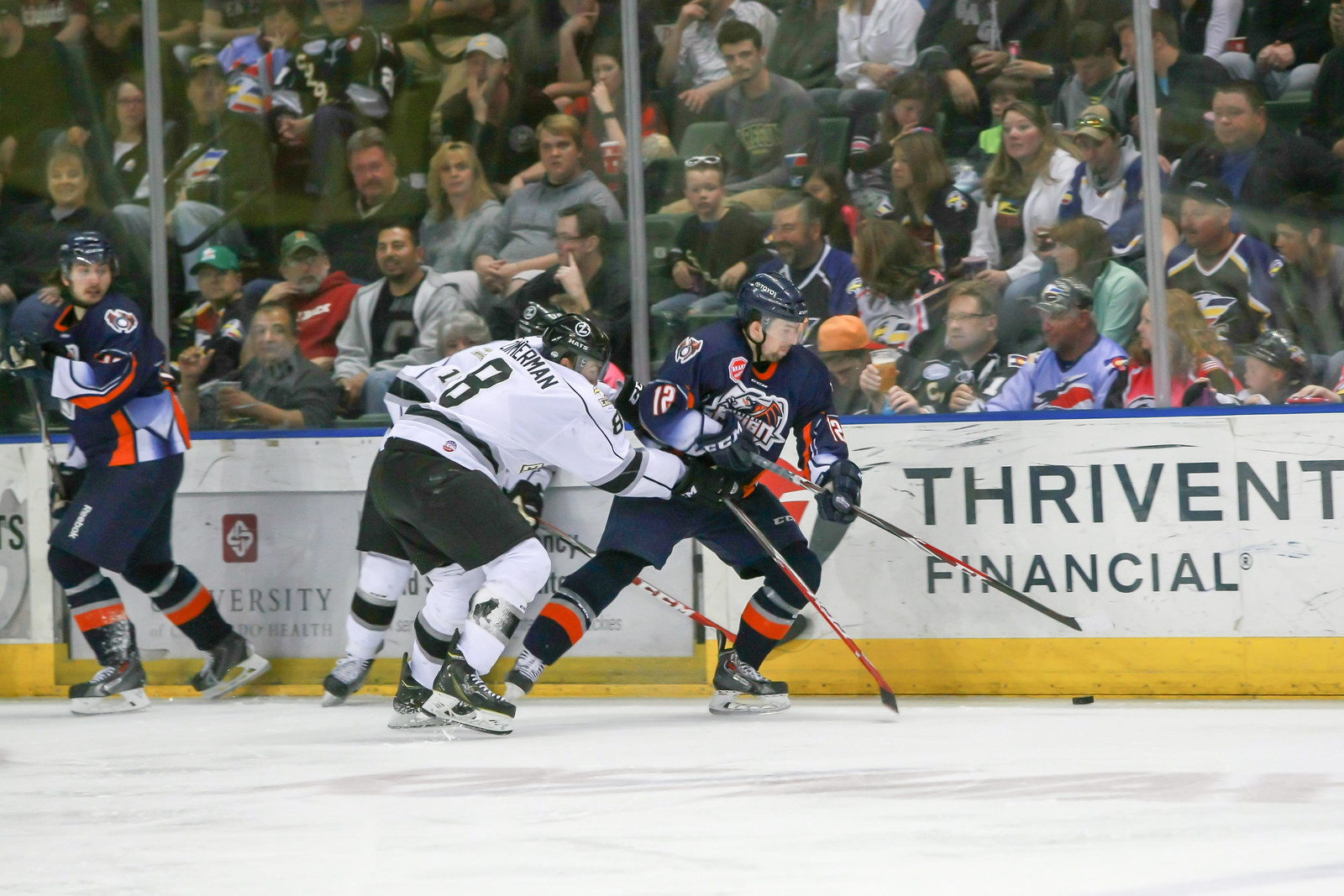This photograph captures an intense moment during a professional hockey game in landscape view. In the center of the image, a player in a dark blue jersey and shorts is seen fighting for the puck with his stick, pursued closely by two opponents in white jerseys and black shorts. Both teams' players are fully geared, including black and blue helmets. On the left side of the frame, another player in dark blue glances back at the action. The rink's border features a distinctive yellow bottom, a white middle section with advertisements, and a red and blue top. The ice rink is surrounded by a plastic barrier, beyond which a lively crowd of diverse fans, including men, women, and children, intently watches the game unfold. The enthusiasm of the spectators is palpable as they react to the fast-paced action on the ice.